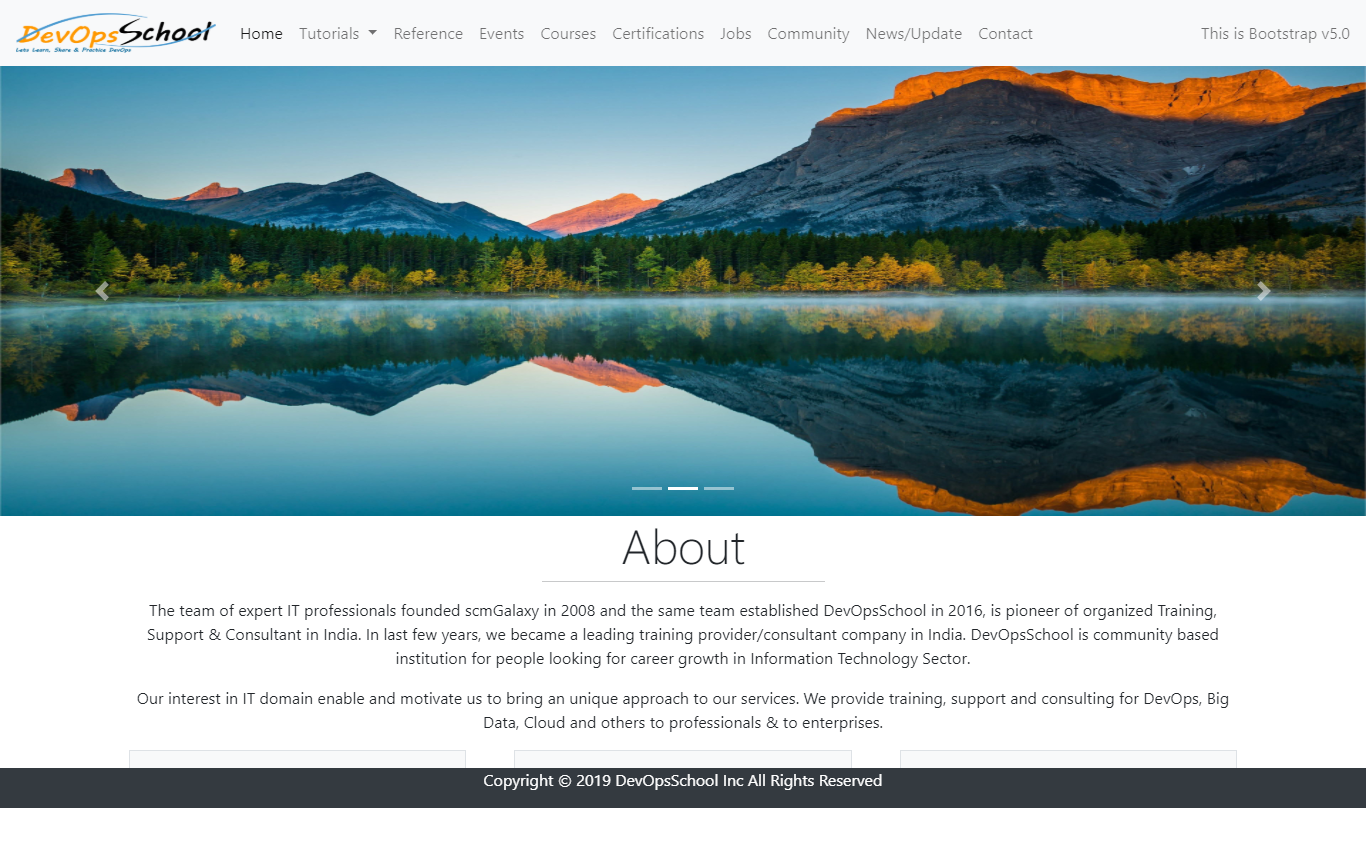## DevOps School Website Snapshot

The image captures a section of the DevOps School website, showcasing its comprehensive navigation menu. The sidebar lists various sections including: Home, Tutorials, Reference, Events, Courses, Certifications, Jobs, Community, News/Update, and Contact. At the top of the page, there's a banner stating "Bootstrap v5.0".

The background features a stunning photograph of a serene lake, surrounded by lush trees at its edges and majestic mountains rising in the distance. The mountains ascend towards the sky, filling most of the picture to the top on the right side, with a sliver of sky visible on the left. This scenic view is perfectly mirrored in the calm waters of the lake below, creating a beautiful, symmetrical reflection.

In the About section below the image, the text details the origins and mission of the institution: "The team of expert IT professionals founded SCM Galaxy in 2008 and established DevOps School in 2016, pioneering organized training, support, and consultancy in India. In the last few years, we have become a leading training provider and consultancy company in India. DevOps School is a community-based institution for those seeking career growth in information technology." The section continues with further elaboration and numerous articles.